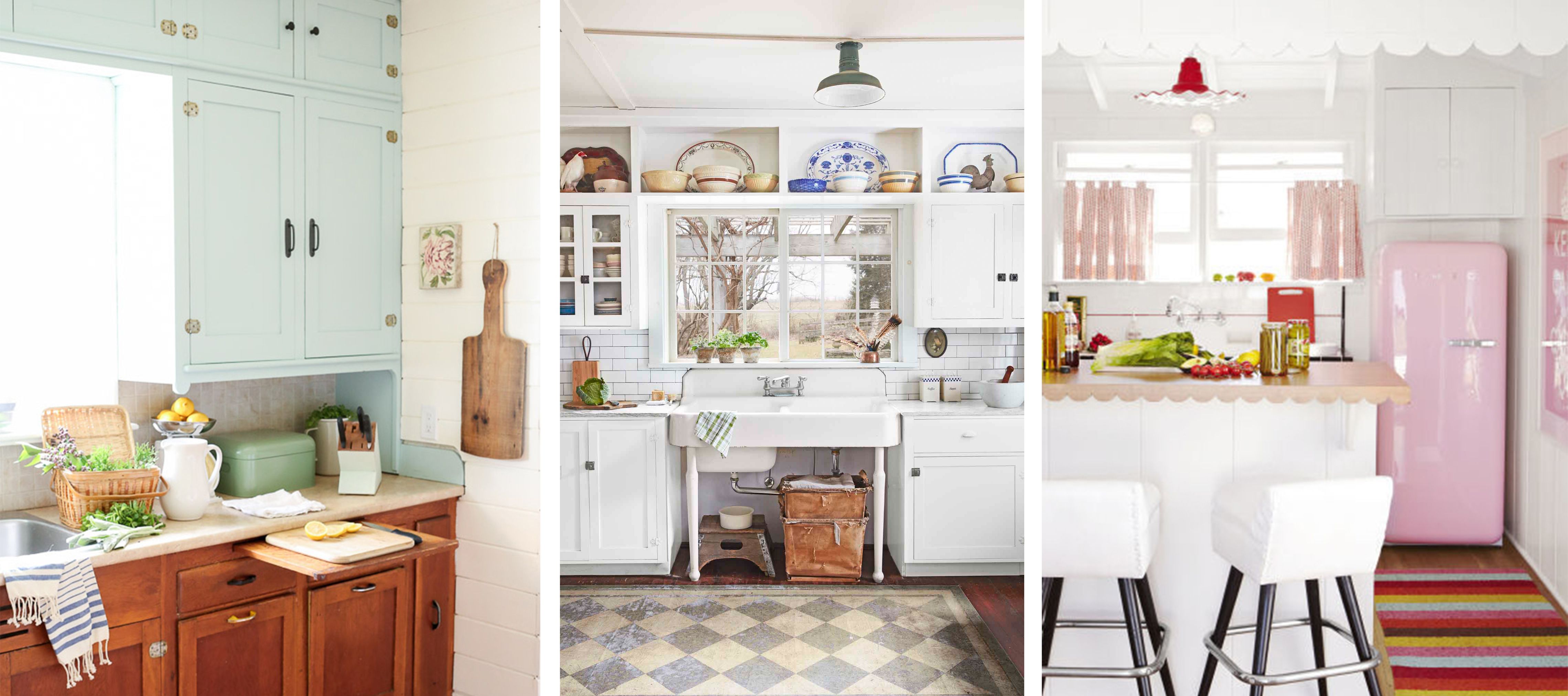The image presents a triptych of side-by-side, equally-sized rectangles, each depicting a unique kitchenette design. 

In the left image, a charming kitchenette is highlighted with blue and brown cabinetry. The upper counter is adorned with a white pitcher, flowers, a recipe box, and a towel, blending functionality and decor. A cutting board hangs on the wall and a small utility shelf is pulled out below the countertop. Stainless steel accents, including a sink, enhance the rustic yet polished aesthetic. Baskets, pitchers, and a knife holder contribute to the country kitchen style.

The central image showcases a more modern kitchen. It features a checkerboard blue and white rug on brown floors, with white cabinets surrounding a sleek, open-legged sink. The backsplash is also white, and the kitchen is lit by barn-style lamps, adding a rustic charm. Above the cabinets, there are areas for displaying pottery and serving dishes, while a multi-pane window above the sink allows natural light to stream in. Leather totes and a step stool are neatly tucked under the sink, accentuating the utilitarian design.

The right image offers a playful, vintage-inspired kitchenette with a striped rug in the bottom right corner. Dominated by light pink tones, the setting includes a white counter with a pink countertop, a small pink refrigerator, and curtains with pink vertical stripes on the windows to the left. A kitchen bar with two white-cushioned stools creates a casual dining area, tying together the whimsical and cozy atmosphere of this eclectic space.